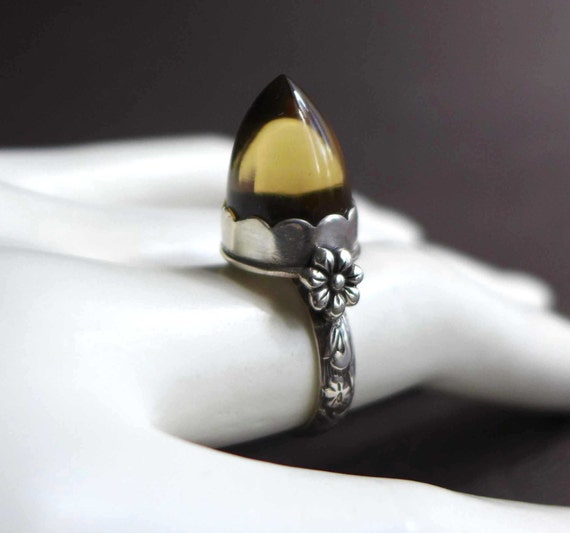The image depicts a highly detailed color photograph of a white mannequin's left hand set against a dark, burgundy-tinged black background. The focus is on the index finger, which is adorned with an ornate silver ring. The ring, which appears slightly tarnished, features intricate floral patterns along the band. At the top, the ring showcases a silver flower with delicate petals surrounding a raised, half-egg-shaped gemstone. The gem is a glossy brown with a striking yellow center, bordered by scalloped silver edges. Light casts shadows onto the mannequin's hand, adding depth and emphasizing the craftsmanship of both the ring and the hand's ceramic-like texture.